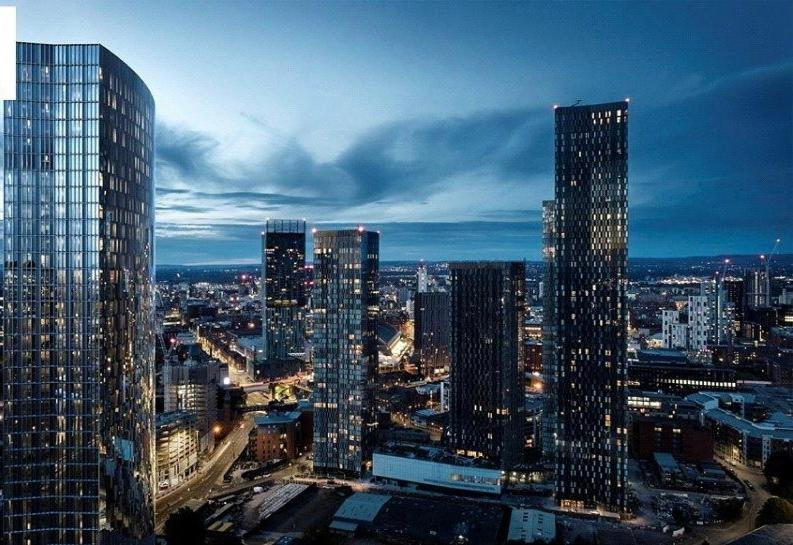This photograph captures an elevated, panoramic view of a bustling urban metropolis during twilight, either early morning or late evening. The city stretches out beneath us, suggesting the image may have been taken from a high vantage point such as a helicopter, drone, or a skyscraper. The skyline is dominated by numerous towering skyscrapers with dark, glassy exteriors that reflect the ambient light. The tallest buildings, while largely dark, glisten with sporadic illuminated windows. Below, the city's roadways weave through the forest of structures, glowing with streetlights that cast a yellowish-orange hue. Smaller, lighter-colored buildings, possibly made of cement or blocks, are scattered especially towards the right-hand side and the bottom center of the image. The sky adds to the scene's atmosphere, transitioning from a lighter blue on the left to a deeper blue on the right, enhanced by clouds. The absence of the sun hints that it has just set or is about to rise, casting a gentle glow across the cityscape and the horizon stretching far into the distance.